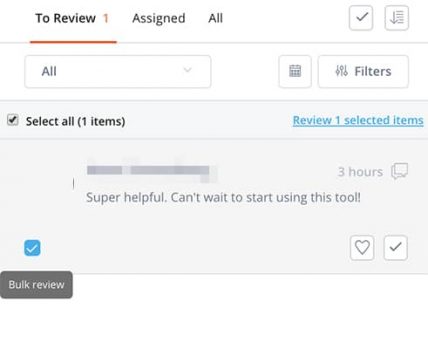This image is a screenshot of the review section of a website. The top left corner features a menu bar with bold black text reading "To Review," accompanied by an orange "1" indicator and an orange horizontal bar below it. To its right are additional menu options labeled "Assigned" and "All" in black text. 

In the top right corner, there are two light gray boxes: one containing a dark gray checkbox and the other featuring a light gray arrow pointing downward alongside horizontal lines. Below the menu bar are three gray option buttons. The leftmost button is a dropdown menu set to "All" in black text, while the two buttons on the right display a calendar icon and the word "Filters," respectively.

At the bottom of the image, a review is displayed in light gray text. The title or author's information is blurred out, but the review itself reads, "Super Helpful. Can't wait to start using this tool," and was written three hours ago. This review appears to be selected, as indicated by a light blue box with a white checkmark in the bottom left corner. 

Additional features include "Select All" in black text with "(1 Items)" in parentheses in the top left corner of the review, and a blue hyperlink in the top right corner stating "Review One Selected Items." Just below the review, in the bottom left, is a dark gray box with white text labeled "Bulk Review."